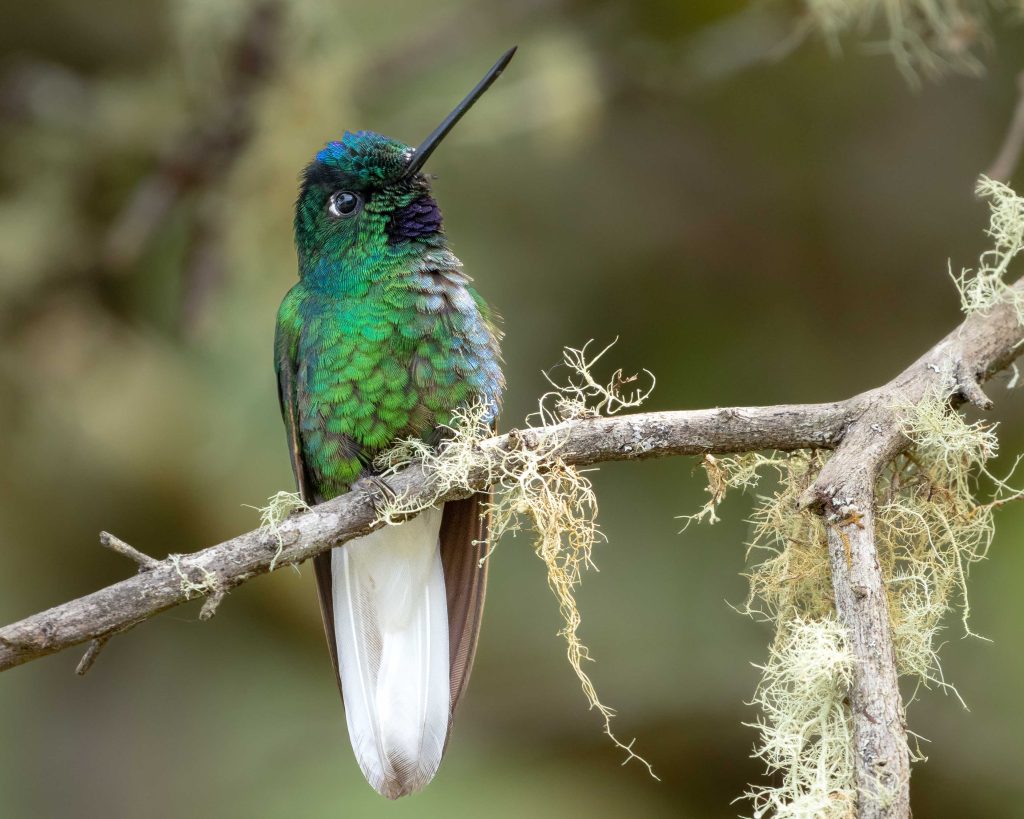This photograph captures a striking emerald-colored hummingbird perched gracefully on a delicate, twiggy branch adorned with light yellowish dried moss. The bird's iridescent feathers shimmer brilliantly, fluffed up to showcase their vibrant colors, especially the intricate details of its black throat and the subtle white patch on its chest that complements the white underside of its tail. The hummingbird's expressive and intense eye adds to its captivating presence, emphasizing its alert demeanor. The focus on its elongated bill highlights the precision and clarity of the image, providing a rare still glimpse of this usually fast-moving creature. The softly blurred background hints at a lush, tree-filled environment, accentuating the natural beauty and tranquility of the scene. Such a precious little guy, this hummingbird embodies elegance and charm, making the photograph truly endearing.